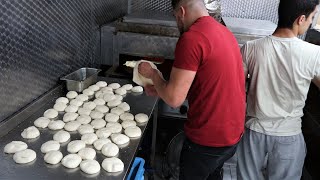This is a detailed color photo of a commercial kitchen scene featuring two individuals working side by side. The man on the left is wearing a red t-shirt and dark pants, and he appears to have a short, faded hairstyle. He is meticulously placing bowls of dough onto a flat top cooking surface, which resembles a griddle commonly found in such kitchens. The dough he is handling looks to be forming biscuit-like shapes. Directly beside him on the right is another man dressed in a white t-shirt and gray sweatpants. This man, who has dark, regular-length hair, is looking away to the right with his back partially turned to the other man. The backdrop of their workspace includes a stainless steel wall adorned with a carbon fiber or diamond diagonal pattern. Additionally, a blue towel or blue tub is visible underneath the cooking surface, along with a container, indicating their utility in the kitchen's operations.